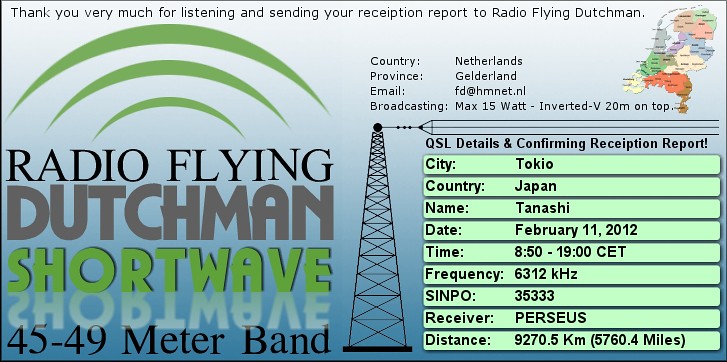The horizontally aligned rectangular image has a thin black border at the top and left-aligned small black text that reads, "Thank you very much for listening and sending your reception report to Radio Flying Dutchman." In the upper right-hand corner, there's a small, illegible map with areas shaded in different colors. On the left side of the image are three curved green lines increasing in size from bottom to top, with text below saying "RADIO FLYING DUTCHMAN SHORTWAVE 45-49 METER BAND." The letters "RADIO FLYING" are in black, "DUTCHMAN" is in grey block letters, and "SHORTWAVE" is in green block letters.

In the middle of the image, there is a black radio tower with text above it stating "Country: Netherlands, Province: Gelderland, Email: fd@hmnet.nl, Broadcasting Max: 15 Watts, Inverted V, 20M on Top." To the right of the radio tower, under the heading "QSL Details and Confirming Reception Report," the following details are provided: "City: Tokyo, Country: Japan, Name: Tanashi, Date: February 11, 2012, Time: 0850 to 1900 CET, Frequency: 6312 kHz, SINPO: 35333, Receiver: Perseus, Distance: 9270.5 kilometers (5760.4 miles)."